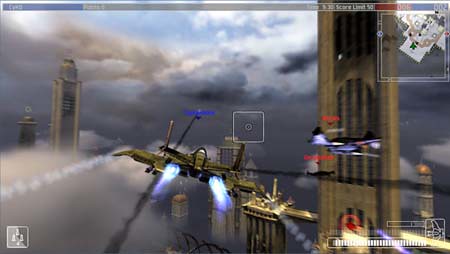This photograph captures a slightly blurry screenshot from a video game featuring a dynamic cityscape setting with towering skyscrapers under a stormy sky. The central figure in the image is a futuristic flying machine resembling an X-Wing fighter from Star Wars, emitting light blue flames and trailing smoke from its rear propellers as it navigates through the cloud-laden atmosphere. The bottom right corner of the screen displays the player's energy or life level, represented by a series of white and light gray rectangles. In the top right corner, a small map shows the player's current location within the game, while the top center of the screen features a score indicator, potentially reading a value such as '50'. The overall color palette of the screenshot includes various shades of white, gray, black, blue, and red, adding to the animated and vibrant feel of the scene.